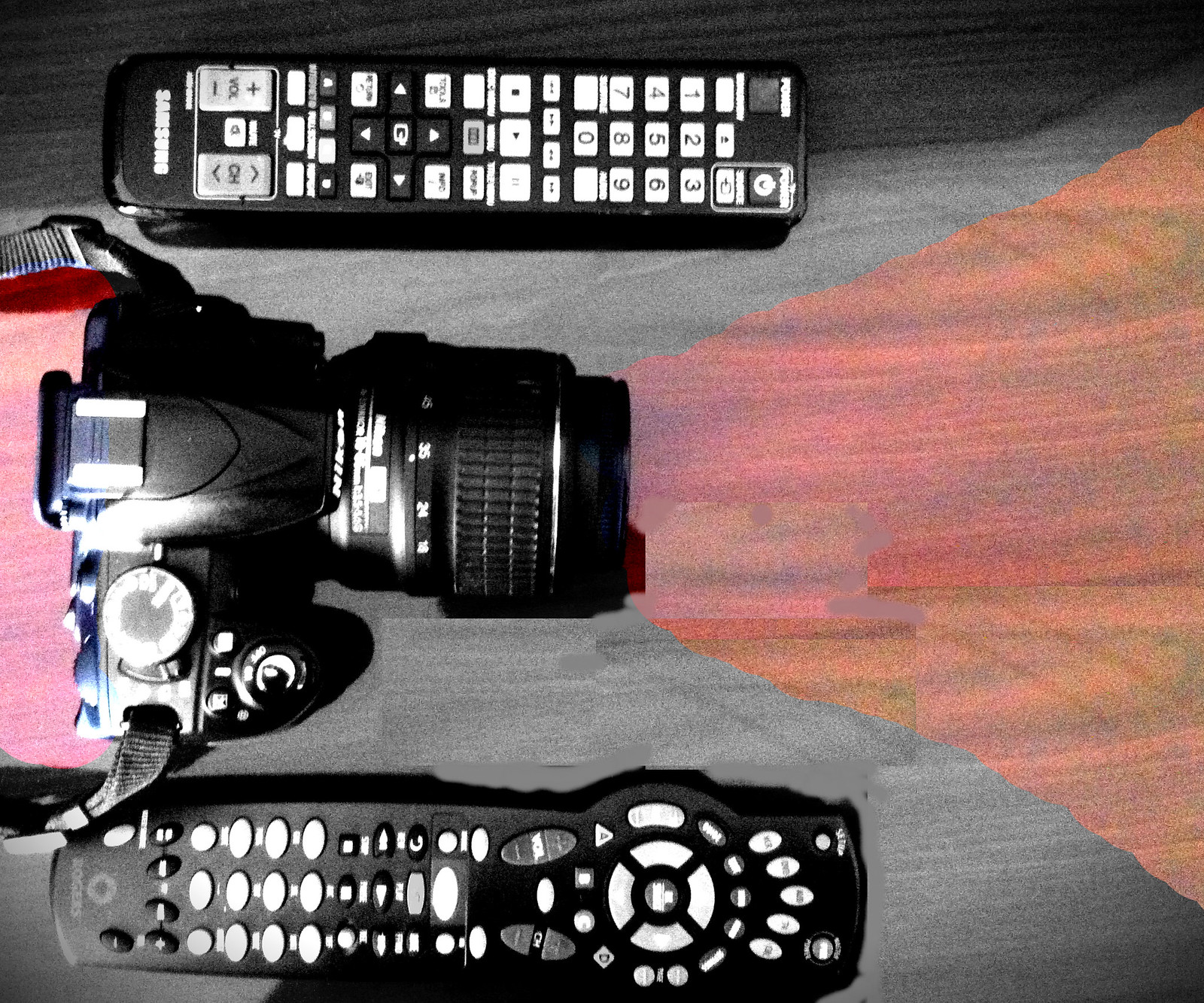This is a black and white photograph featuring a high-tech Nikon DSLR camera positioned between two TV-style remote controls. The photograph, taken from an overhead perspective at about a foot above, captures the scene on a wooden surface that exhibits an intricate pattern of black and brown wood, including a visible diamond and triangle design. The camera, centered in the image with its large lens pointing to the right, contrasts against the varied wood tones. Above the camera is a Samsung remote, identifiable by its logo, and below it lies a slightly larger unidentified remote. Both remotes are adorned with a plethora of buttons, numbering between 30 and 40, and display a mix of white and gray buttons. The edges of the image subtly reveal the original color tones of the wood, hinting at the photograph's transformation from color to black and white.